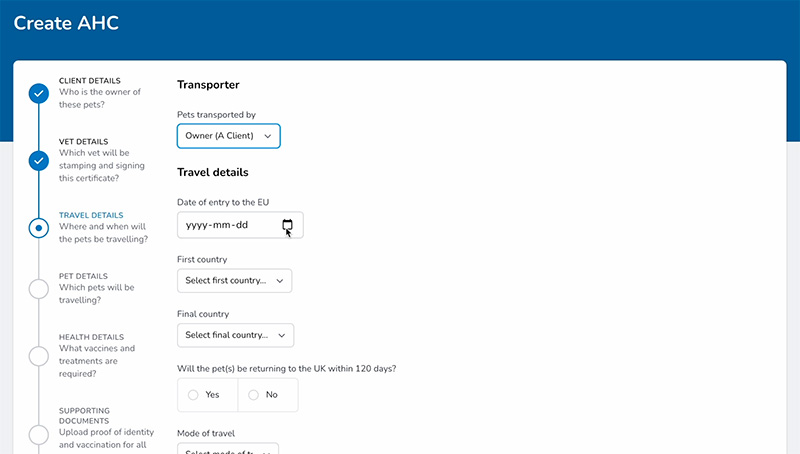**Title: "CREATE AHC"**

In the upper left-hand corner of the image, the title "CREATE AHC" is displayed prominently in white font. The letters "A H C" are capitalized, while the word "Create" starts with a capital "C." 

The main feature of this interface is a vertical status bar positioned in the center. The status bar consists of multiple sections, each representing different steps and information categories. 

1. **Client Details:** The first section, labeled "Client Details," is checked off, indicating that the information about the owner of the pets has been completed.
   
2. **Vet Details:** The second section, "Vet Details," is also checked off, confirming that the veterinary information has been provided.

3. **Travel Dates:** The third section is currently active, suggesting that users are currently inputting or verifying the travel dates for the pets.

4. **Pet Details:** The fourth section is labeled "Pet Details," awaiting completion.

5. **Health Details:** The fifth section, "Health Details," also awaits completion.

6. **Supporting Documents:** The final section on the vertical status bar is "Supporting Documents," which remains incomplete.

To the right of the status bar, another vertical menu offers additional navigation options, starting with "Transporter." This layout ensures users can efficiently progress through the various steps needed for the process, with clear indications of what has been completed and what is still pending.

The user interface is well-organized for ease of use, ensuring that all necessary details for creating an AHC (Animal Health Certificate) are methodically addressed.